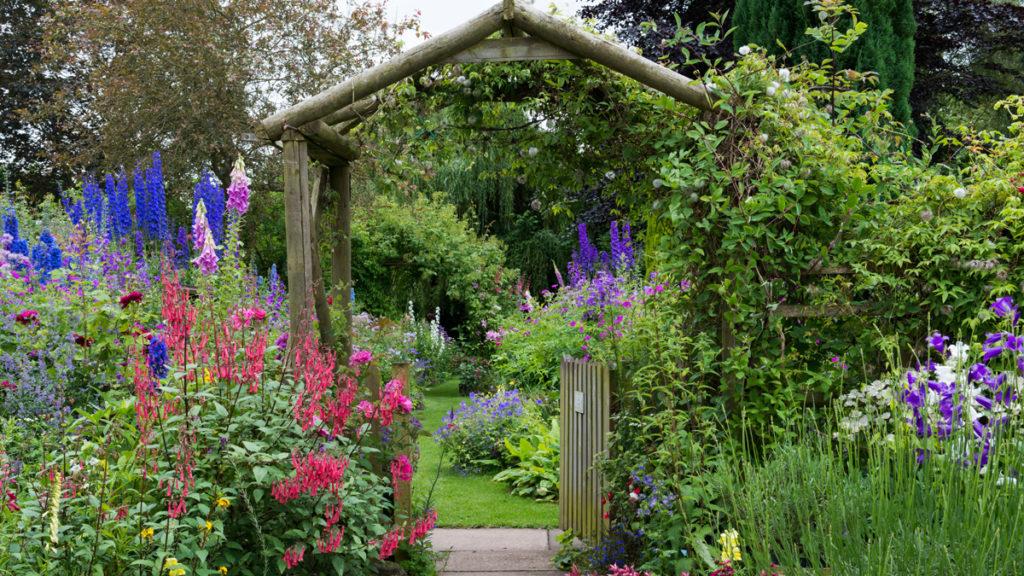The image is a color photograph of a lush and densely packed garden, showcasing a diverse array of vibrant flowers in shades of blue, purple, pink, white, red, yellow, indigo, and magenta. Central to the composition is a prominent wooden archway or trellis, framed by an open wooden gate that invites entry into the garden. The garden's vegetation appears abundant and slightly overgrown, with tall flowers and rich green leaves suggesting meticulous care. To the right of the trellis, vegetation grows profusely along its sides, adding to the garden's wild charm. Behind the flowers, thick bushes and trees form a verdant backdrop. The notable flowers on the right side include purple, white, and tall grass, while the left side features a mix of pink and blue flowers. The predominant color throughout the scene is green, creating a vivid contrast with the diverse and colorful blooms scattered throughout the garden.